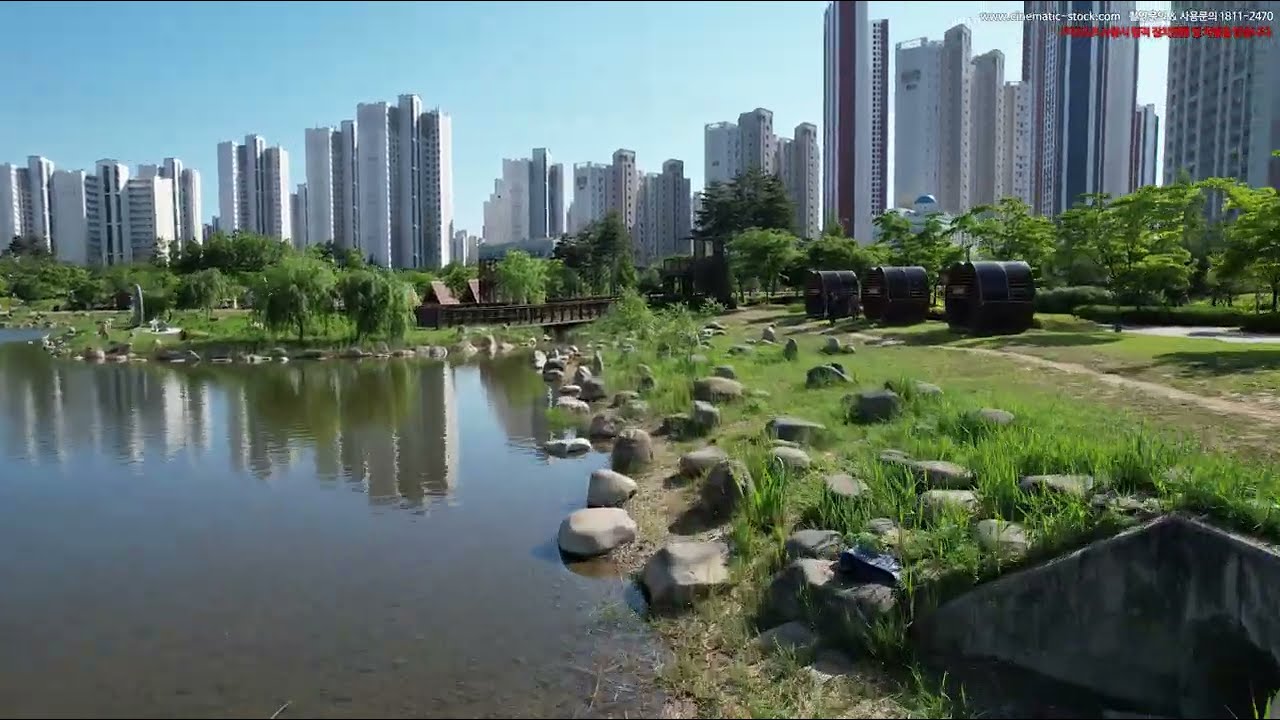In the foreground of the image, there is a serene water body, its surface calm and reflecting a congregation of tall skyscrapers that dominate the upper portion of the frame. These multistory buildings, primarily painted white, exhibit hints of maroon and blue stripes, and some feature large glass windows. The structures rise up against a backdrop of a vivid blue sky. 

The bottom left of the image is particularly striking, showcasing a collection of cylindrical, black structures resembling giant hamster wheels. There are three of these unusual forms stationed near the water’s edge, aligned along a path. Surrounding the shoreline and interspersed throughout the lower portion of the scene are an array of clean white boulders and rocks. Their seemingly deliberate arrangement gives off an artistic, almost surreal quality, further enhanced by the presence of short trees with green foliage scattered throughout the area. 

In the top right corner of the image, there is some white and red writing, though its details are indistinct. Additional writing appears on several of the skyscrapers, possibly indicating the names of the buildings’ occupants. Overall, the composition melds natural and urban elements, creating a fascinating juxtaposition of the real and the surreal.